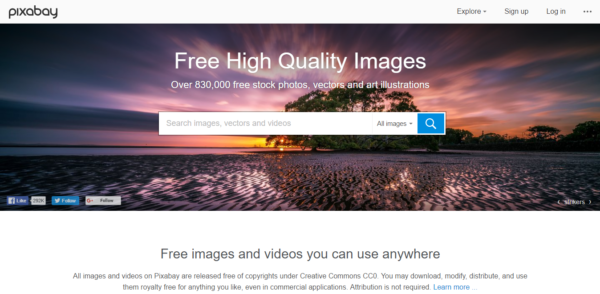This screenshot from the Pixabay website showcases its extensive offering of high-quality, free stock photos, vectors, and art illustrations. The top left corner prominently displays the Pixabay logo, indicating the site's branding. To the right, a navigational menu offers options such as 'Explore,' which is expandable, 'Sign Up,' 'Login,' and an ellipsis for additional features.

The centerpiece of the screenshot is a rectangular image featuring a beautifully vibrant scene of trees, adorned with hues of pinks, purples, golds, and reds, underscoring the high quality of the images available on the platform. A faint watermark is visible at the bottom right of the image, though it is not entirely legible. Below this, white text announces, "Free high-quality images: over 830,000 free stock photos, vectors, and art illustrations."

A search box allows users to search for images, vectors, and videos, with a drop-down to refine the search categories and an adjacent blue magnifying glass icon to initiate the search.

Social media buttons are positioned at the bottom left, providing options to like the page on Facebook, follow on Twitter (or X), and follow on Google Plus. Beneath these buttons, text emphasizes the terms of use for the site, stating, "Free images and videos you can use anywhere. All images and videos on Pixabay are released free of copyrights under Creative Commons CCO. You may download, modify, distribute, and use them royalty-free for anything you like, even in commercial applications. Attribution is not required." A 'Learn More' link provides additional information, confirming that all resources on the site are entirely free and unrestricted by copyright requirements.